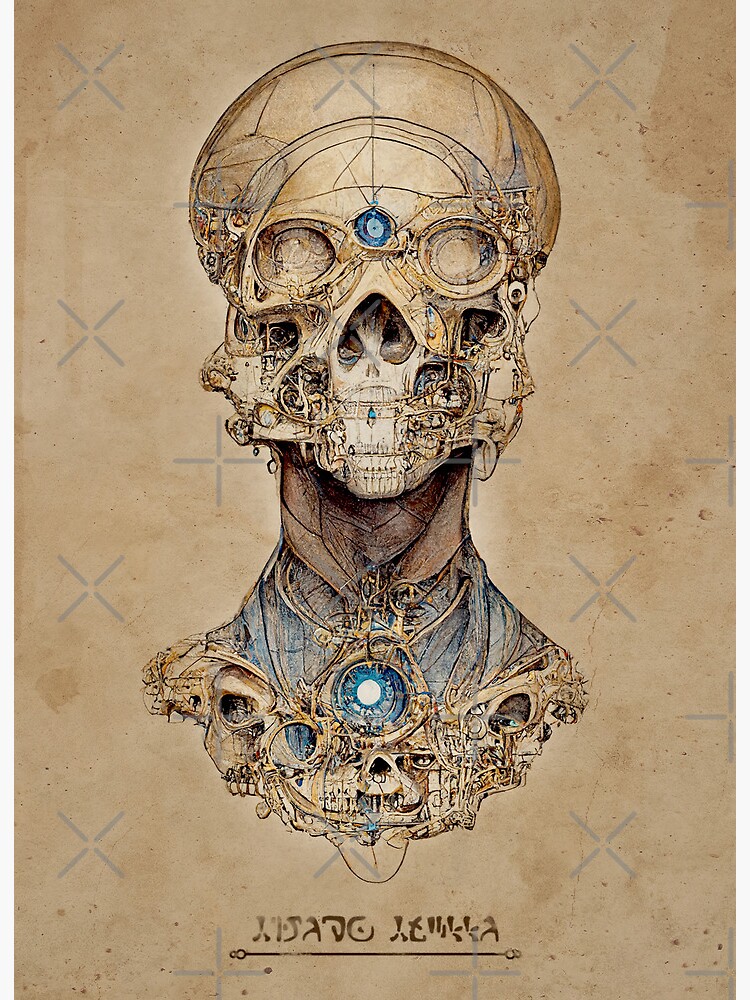The image is a detailed, steampunk-inspired illustration on a tan, aged paper-like background, peppered with light watermark "X"s in a grid pattern. The central figure is a human skull with intricate gears and mechanical elements inside and around it, blending bone and steampunk aesthetics. The skull is decorated with blue jewels embedded in the forehead and the upper chest area, just below the Adam’s apple. The neck appears realistic, transitioning into a blue Nehru-collared tunic adorned with skeletal and mechanical motifs. The lower part of the image features a line of enigmatic text in a language resembling Arabic, underlined by a brown line with small circles at each end. The entire artwork is a blend of pencil and ink, combining elements of futuristic technology and classical anatomy.